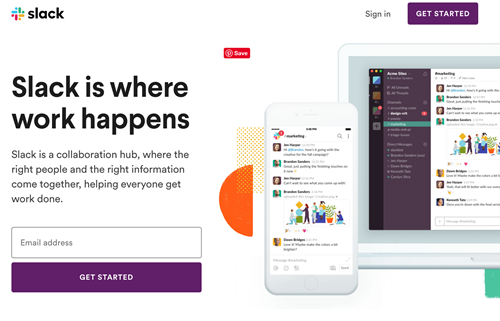**Caption:**

This screenshot from a website features the Slack homepage. The image has a predominantly white background. In the top left corner, the Slack logo is displayed in black text adjacent to a multicolored symbol comprising blue, green, red, and yellow elements. On the right side of the header, a "Sign In" button and a "Get Started" button in purple with white text are visible.

Centralized on the left side, the bold black text reads "Slack is where work happens." Below this, additional text describes Slack as "a collaborative hub where the right people and the right information come together, helping everyone to get work done." Midway down, there's an input box for an email address and another purple "Get Started" button. A red "Save" button appears in the middle, though its purpose is unclear.

On the right side of the page, there's an image depicting both a mobile phone and part of a desktop screen, suggesting the multi-platform functionality of Slack. Beside the devices, a decorative yellow rectangle with yellow dots and a half-circle in orangey-red adds a splash of color. The mobile phone screen appears to show a list of messages, which is partly mirrored on the laptop screen. The laptop also displays a sidebar with a purple background and white text, with one line highlighted in green. This sidebar includes square icons, adding to the organized layout of the interface.

Overall, the cartoon-like icons and infographics of people enhance the visual appeal and clarity of the collaborative messaging platform's interface.